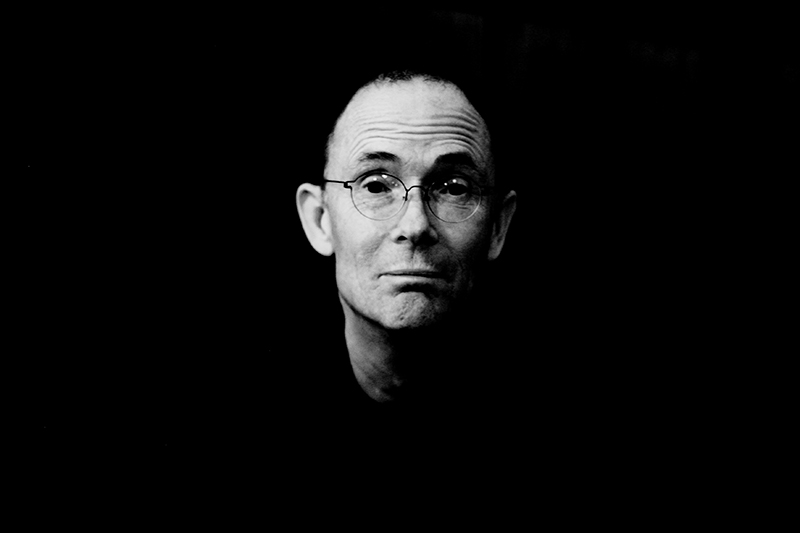In this stark black and white image, an old man, possibly in his 50s, is captured against a completely black background. His face, partially disembodied by the darkness, features prominent Harry Potter-style thin-framed glasses resting on a rigid-looking nose. His slightly raised eyebrows lend a faintly amused and contemplative expression to his wrinkled forehead. Despite the thin, almost emaciated appearance, there's a hint of confidence in his neutral stare. His features include pointy tall ears, a bald or nearly hairless head, and distinct dimples on either side of his nose. Thin eyebrows and a wrinkly chin add to the detailed visage. A small scar, consisting of two lines, is barely visible on the bottom left of his neck. This dramatic, artistic shot evokes the kind of imagery reminiscent of a musician or composer commonly found on the back of an album cover.